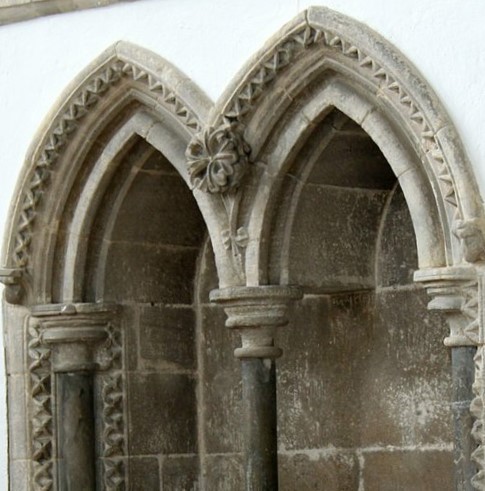The photograph is a close-up of an ornate architectural structure, likely an archway from a historical building such as a church or an old university. The exterior, predominantly off-white, is made of concrete and stone. It features two pointed arches adorned with a repeating pattern along their edges that create a scalloped effect. Within the arches, the stone shifts to a darker grey, suggesting replacement tiles providing foundational support. The archway is structured by three vertically aligned pillars, one central and one on each side, dark grey in color. At the apex of the arches is a decorative element resembling a flower or bow, adding to the intricate ornamentation of the facade. This ornate structure emerges from the wall, leading into an outdoor alcove, and the photograph captures approximately the top half of this detailed design.